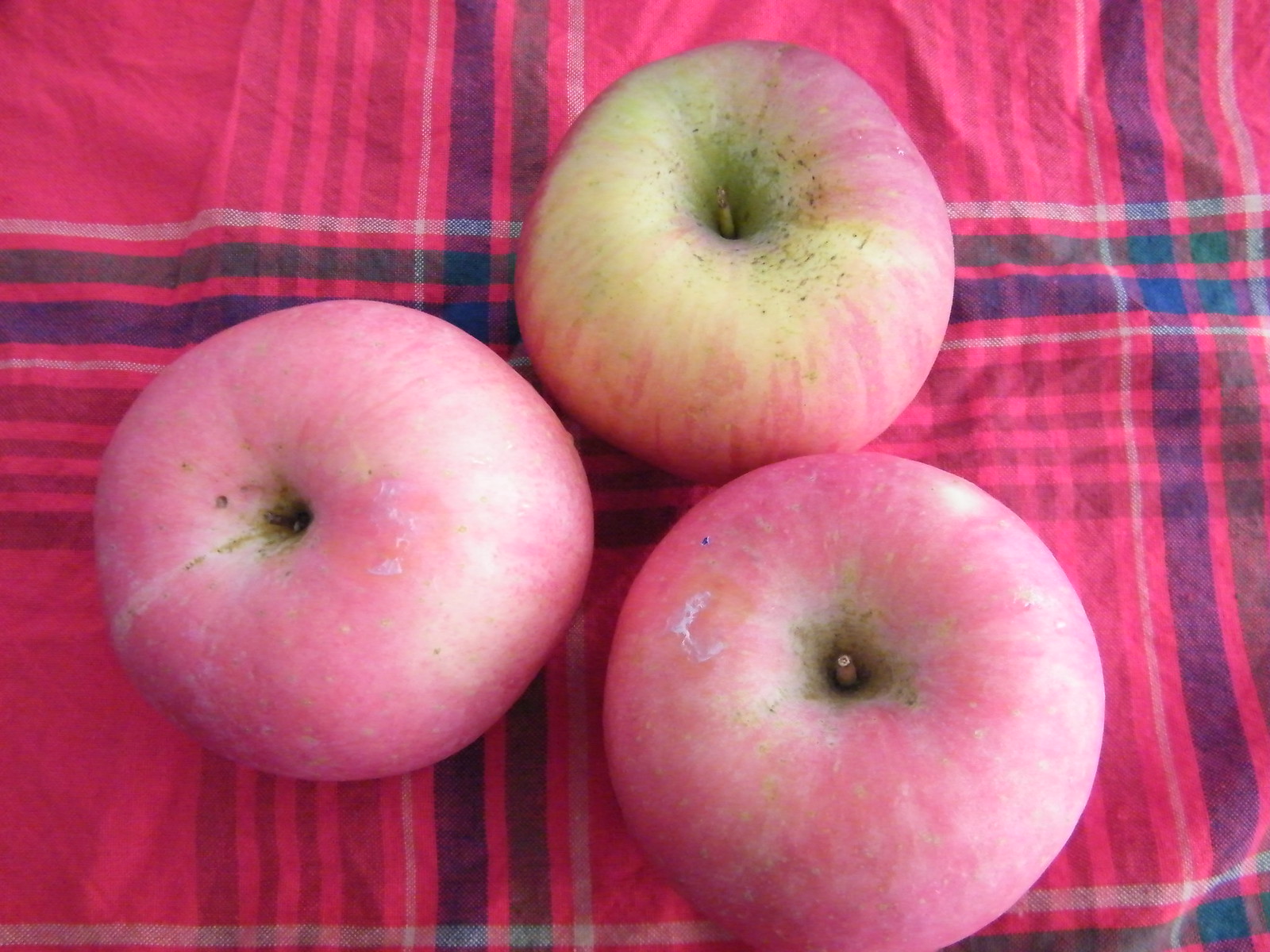A photograph captures three pinkish apples positioned in a triangular pattern on a red and blue plaid cloth, possibly a tablecloth or a blanket. The plaid design features a criss-cross pattern of blue, red, and white stripes, resembling a kilt. The bottom left and bottom right apples appear fully ripe and pink, with one missing its stem. The top apple, less ripe than the others, showcases green hues mixed in with its pink coloration. Each apple reflects a bit of light, giving them a natural, slightly dirty look that enhances their organic appeal. The intricate detailing of the cloth with alternating vertical and horizontal lines adds texture and depth to the image, accentuating the vibrant color contrast between the apples and the background.